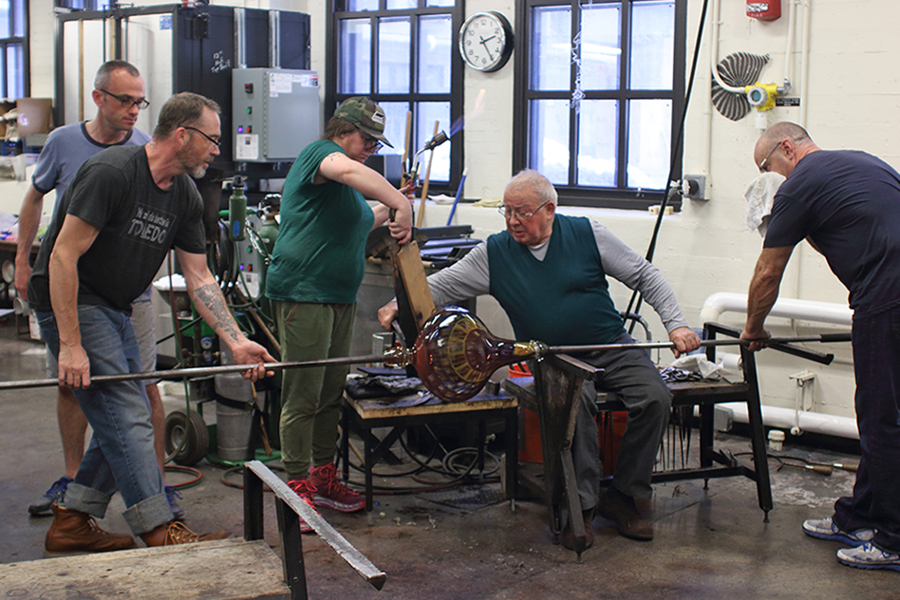In an indoor workshop filled with industrial equipment like compressors, tubes, wires, and an electrical box, a group of people are deeply engrossed in the intricate process of glassblowing. Central to the scene is a middle-aged man wearing a turquoise blue vest over white sleeves. Seated firmly, he expertly manipulates a large, molten glass orb, which displays vibrant hues of purple, red, yellow, and brown. He holds the metal rod steady as he works with precision.

To his left, a woman in a turquoise blue shirt and green pants, sporting a camouflage hat, uses a wooden piece to press against the spinning glass, aiding in its shaping. Nearby, another man in a black shirt and jeans assists by holding the other end of the rod, a white towel in his right hand poised over his mouth. A fourth individual stands back, surveying the meticulous effort. The setting, flanked by white brick walls and adorned with black-framed windows, includes a clock between the windows displaying the time as 2:25. The atmosphere is charged with focus and collaboration, capturing the essence of this traditional craft.